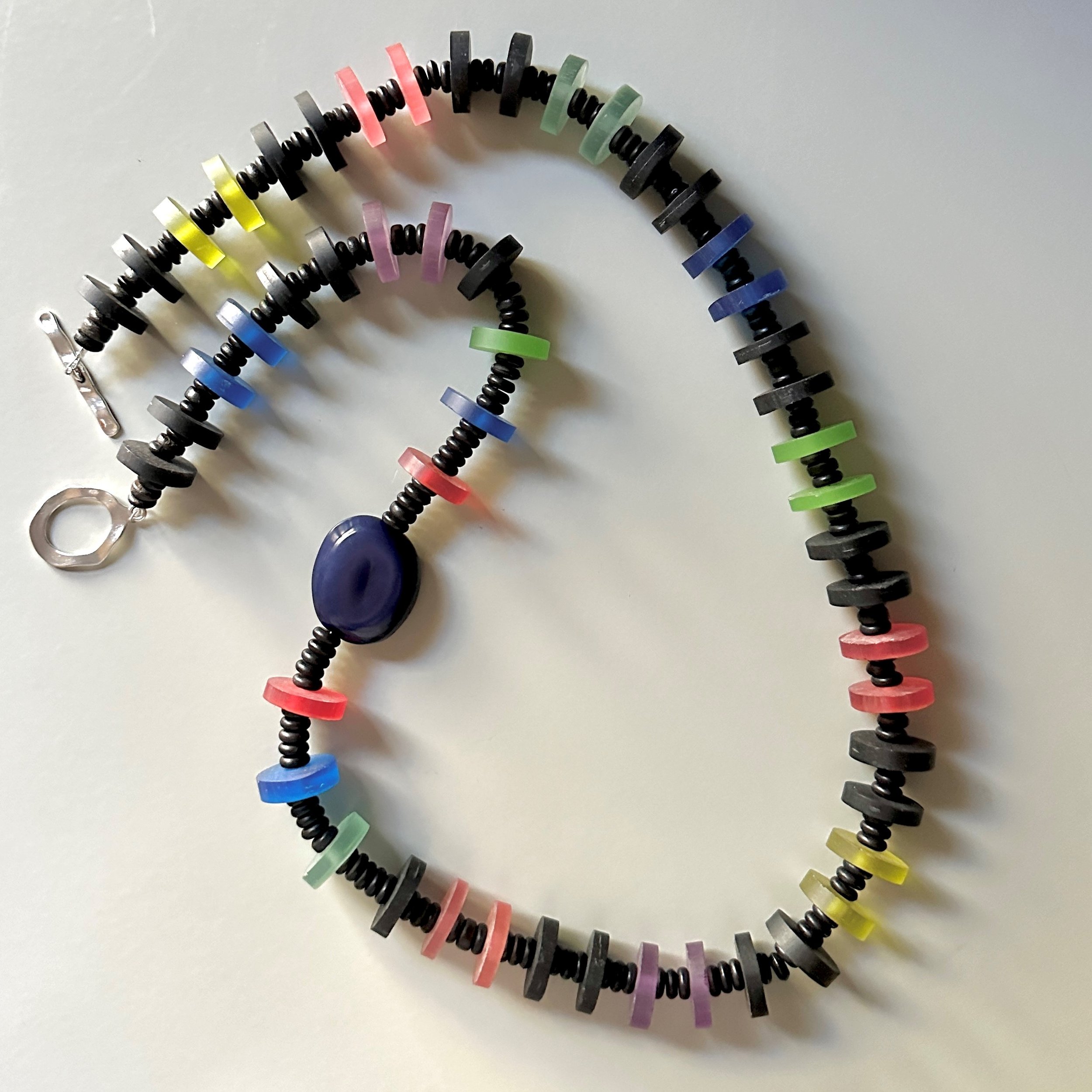The image showcases a handmade beaded necklace laid on a white background that casts noticeable shadows. This long necklace primarily consists of black glass seed beads used as spacers, interspersed with brightly colored rondelle or disc-shaped beads, which appear to be glass but may also be plastic. These decorative beads come in an array of colors, including blue, red, green, seafoam green, pink, gray, purple, and yellow. The colored rondelles are arranged mostly in pairs of the same color, separated by a few black seed beads, before another pair of a different color appears. Toward one end, there's an unexpected large, flattened oval bead that stands out from the rest. The necklace is finished with a toggle clasp, featuring a loop and a bar that fit into each other. The entire piece is illuminated from left to right, highlighting its intricate details and creating a dramatic effect.